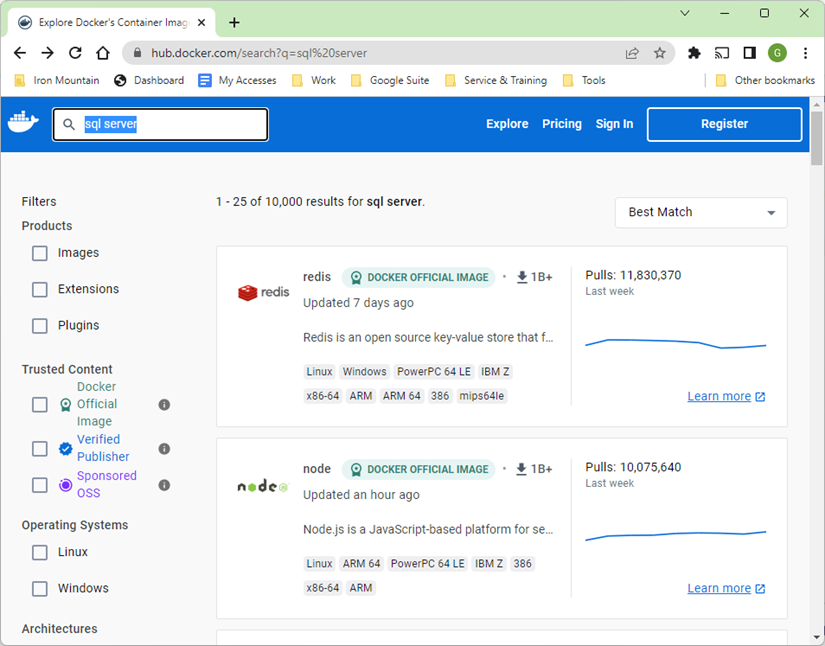This screenshot features a user interface on a web application with a clean white background. At the very top, there's a light green rectangular header. On the left side, there is an open white tab labeled with partially visible options: "Explore," "Dockers," "Container," and "IMAG," with the rest being cut off. The tab also features a logo on the left and an 'X' for closing on the right. Adjacent to this tab, there's a black plus sign.

In the upper right corner of the interface, there are several symbols: a down arrow resembling a lowercase 'v', a dash, a black-outlined square, and another 'X'. Directly below this row, there is another segment featuring left and right navigation arrows, a reload button, a home icon, and a gray search bar where the text "hub.docker.com search" is visible. On the right side of the search bar, there are export and star icons, followed by four additional icons.

Beneath these elements, a list of bookmarks can be found. Below the bookmarks is a prominent blue rectangle, which includes a white logo shaped like a whale with cubes stacked on its back on the left. A large, square search bar is centered within this blue rectangle, displaying the text "SQL Server" in white next to a magnifying glass icon.

To the right within this blue rectangle, the words "explore," "pricing," "sign in," and a "register" button are displayed in white text. Moving down, the interface splits into two sections: the right-hand side contains two graphs, while the left side features filters and product categories including images, extensions, and plugins with corresponding checkboxes. Below these filters, there are additional categories labeled "trusted content," "operating system," and an incomplete view of "architectures."